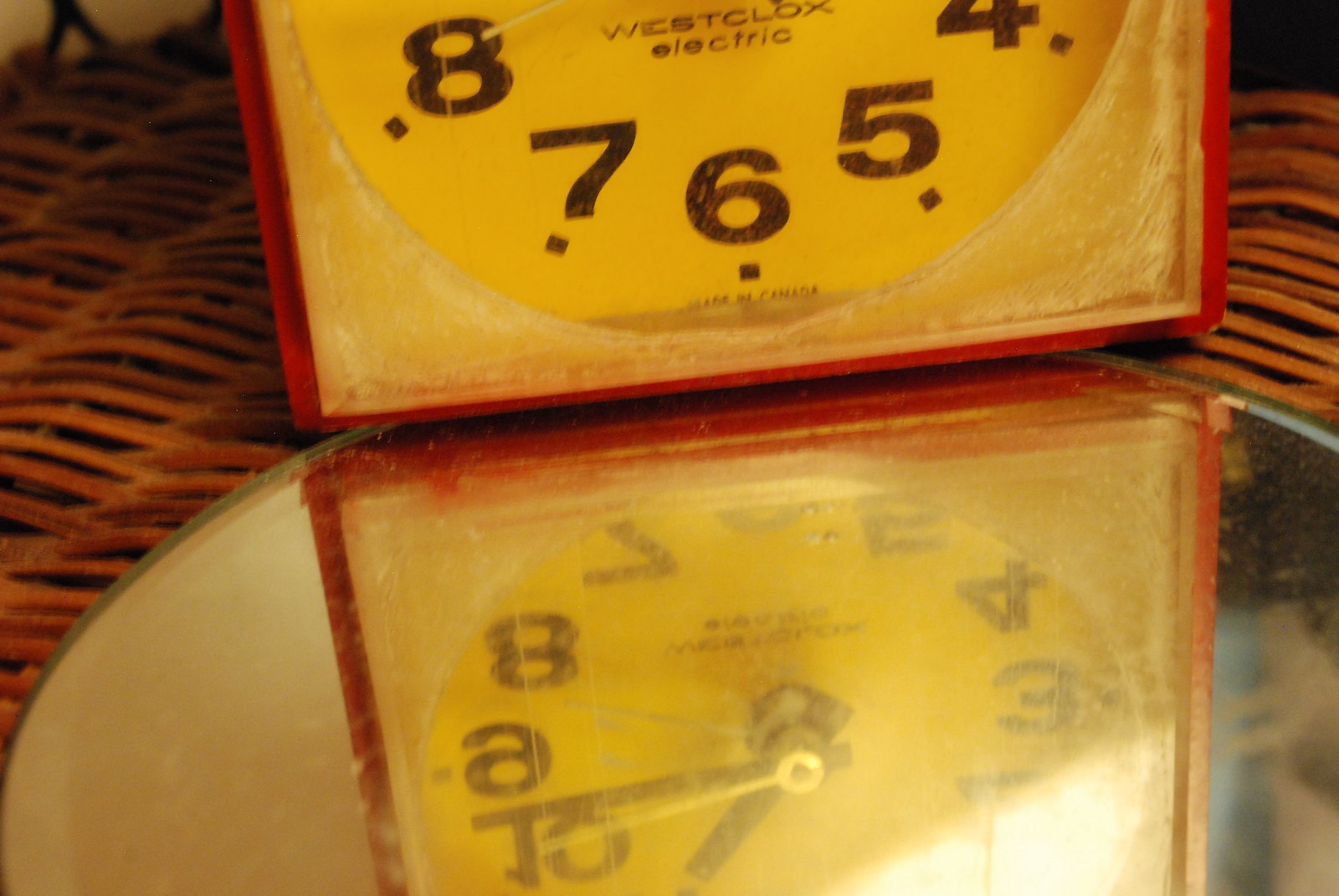The image showcases a detailed composition featuring a square-shaped vintage alarm clock with a reddish-brown outer border and a mustard-colored, round clock face encircled by black numerals, partially visible as 4, 5, 6, 7, and 8. The clock bears the inscription "West Clocks Electric" on the face. The clock is positioned atop a sleek, round mirror that reflects the clock face and hands, capturing the intricate details of the timepiece, including its black and gold hands. The entire setup rests on a background of woven brown fibers, giving it a rustic look, possibly a bamboo or wicker basket, offering a rich, textured backdrop that enhances the visual appeal of the photograph.